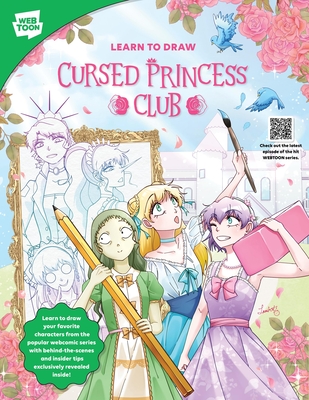The cover of the drawing book titled "Learn to Draw Cursed Princess Club" features a colorful and detailed design. At the top, in three lines of pink letters, the title is prominently displayed. The corners of the cover are adorned with flowers, framing the central artwork. At either side of the word "Club," there are solid pink and outlined pink roses.

The central image showcases three princesses, each holding different art materials. The princess on the left is dressed in a green dress, has greenish skin and small irises, and is holding an oversized pencil pointed upward with both hands. The middle princess, in a bluish dress, is blonde and is shown holding up a pink paintbrush. On the right, a princess with purple hair and blue eyes is dressed in a purple dress with a bow, and is holding a large pink eraser propped against her head. The background behind them features an outline of additional characters with colorful outlines.

Near the top, there's text in a green space that reads, "Learn to Draw Your Favorite Characters from the Popular Webcomic Series with behind the scenes and insider tips exclusively revealed inside." Additionally, a QR code near the bottom invites readers to "Check out the latest episodes of the hit webtoon series."

The overall cover is vibrant and inviting, emphasizing the drawing aspect with the inclusion of large art tools and the colorful framing flowers.